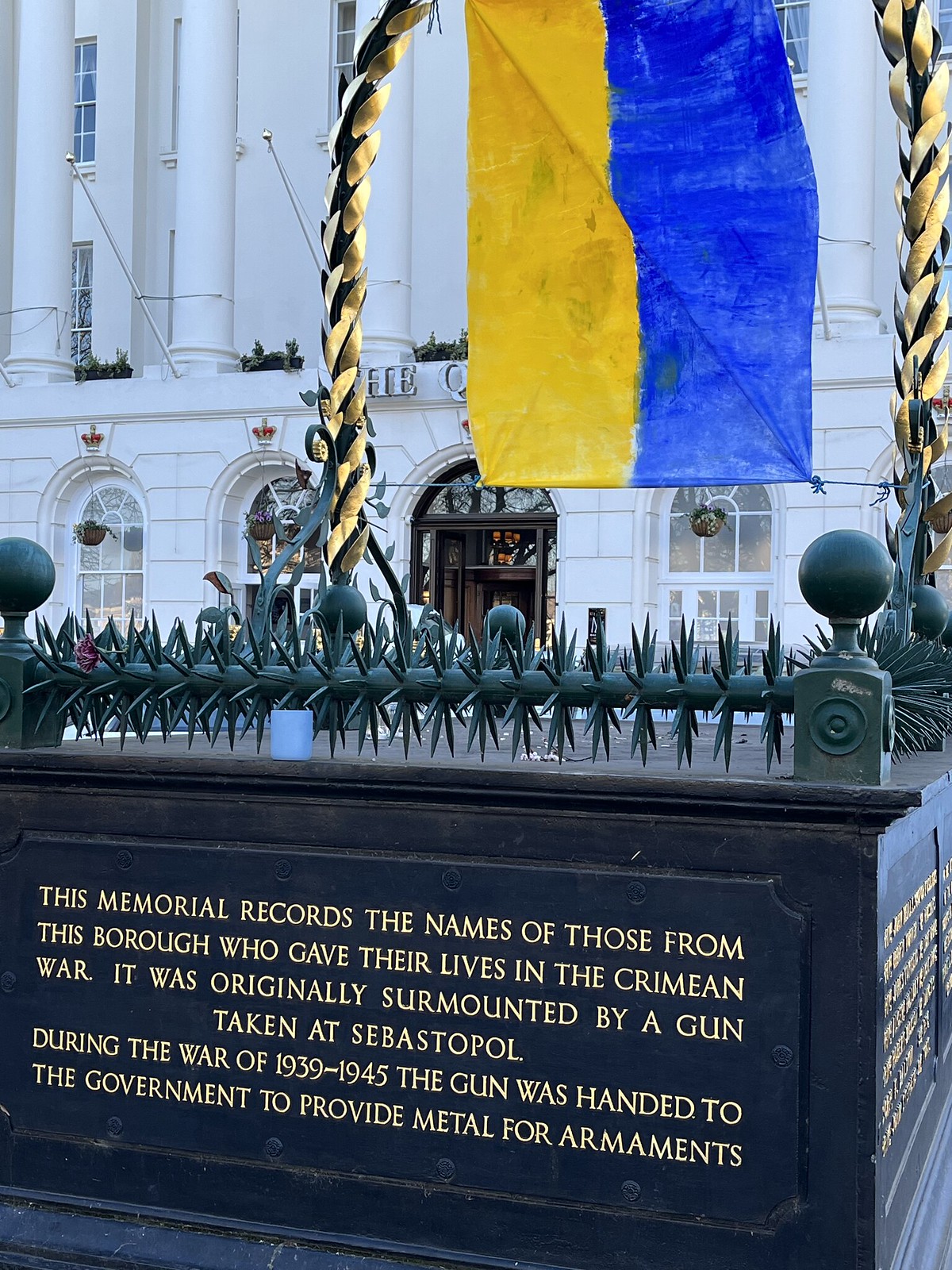In this outdoor daytime photograph, the central focus is a blackish-brown rectangular monument, possibly made of metal or stone. The monument's four corners feature small, raised edges capped with round, bluish-tinged globes. Atop the monument lies a cylindrical metal beam adorned with 360-degree rows of sharp spikes. The front of the monument bears a gold-inscribed plaque that reads: "This memorial records the names of those from this borough who gave their lives in the Crimean War. It was originally surmounted by a gun taken at Sebastopol during the War of 1939 to 1945. The gun was handed to the government to provide metal for armament."

In the background looms a tall, white stone building characterized by its large, white columns starting from the second floor. These columns frame arched doorways and windows, adding to the structure's grandeur. Further enriching the scene, a golden arch with intertwining metalwork resembling twisted vines stands prominently. Dangling from the center of this arch is the yellow and blue flag of Ukraine, symbolizing a poignant connection to heritage and history.